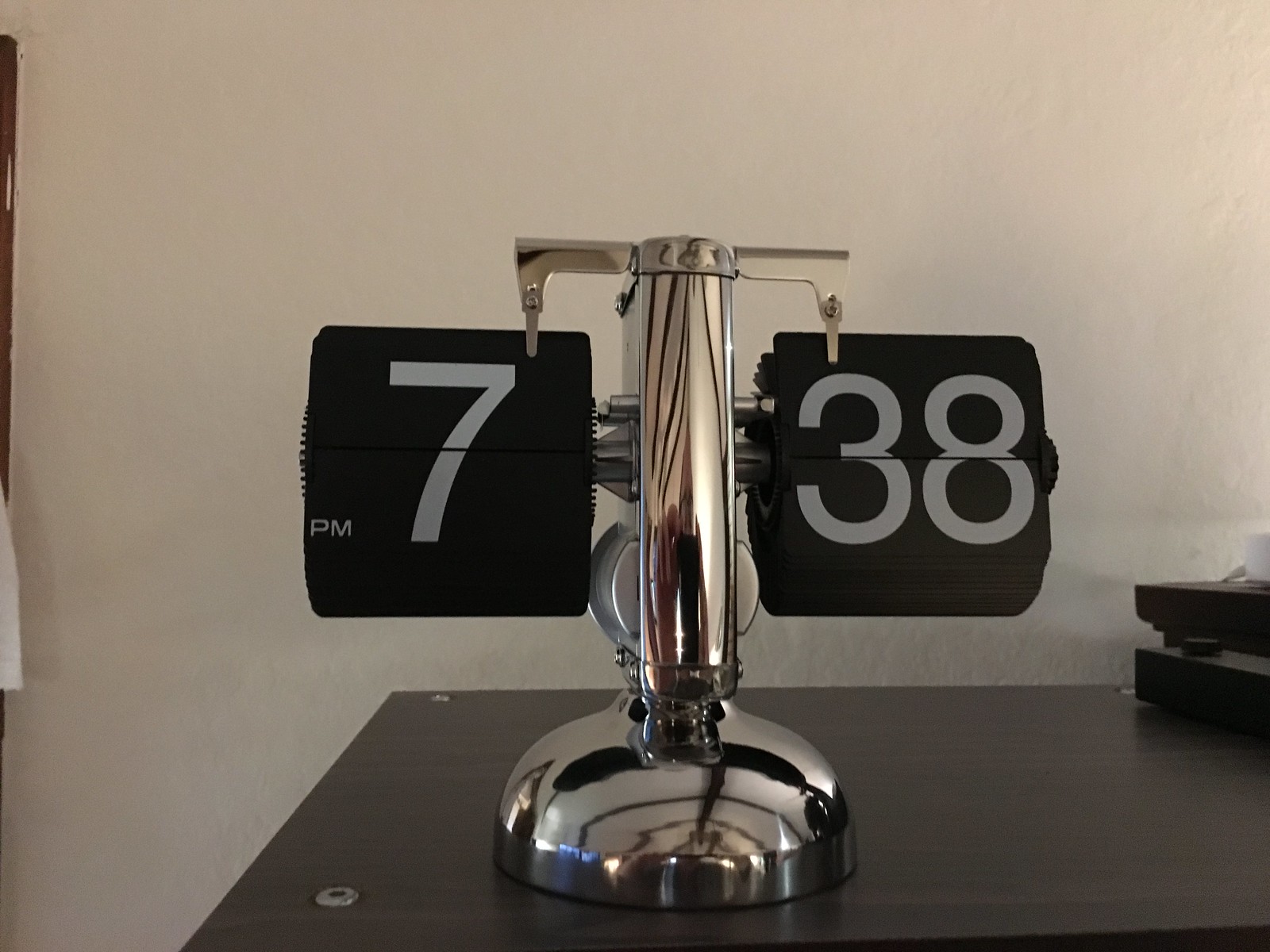This interior image, taken with low, soft lighting, features a desk prominently positioned against a textured, white or off-white wall that shows various imperfections and some bubbling. The desk is a dark cherry wood and showcases a silver vintage-style flip clock centrally placed, designed to display the time. The clock has a shiny silver base and a large center beam extending upward, which branches into two small arms with alligator clips dangling down. The left arm shows an hour card that reads "7 PM" in white text on a black background, while the right arm displays the minute card "38" in similar fashion. Additional details include the presence of two pull-out drawers in the desk's lower right corner and visible silver screws in the corners, suggesting a sturdy construction. In the background, a brown strip with a bit of white can be seen hanging down from the top left, adding to the room's textured and somewhat aged aesthetic.